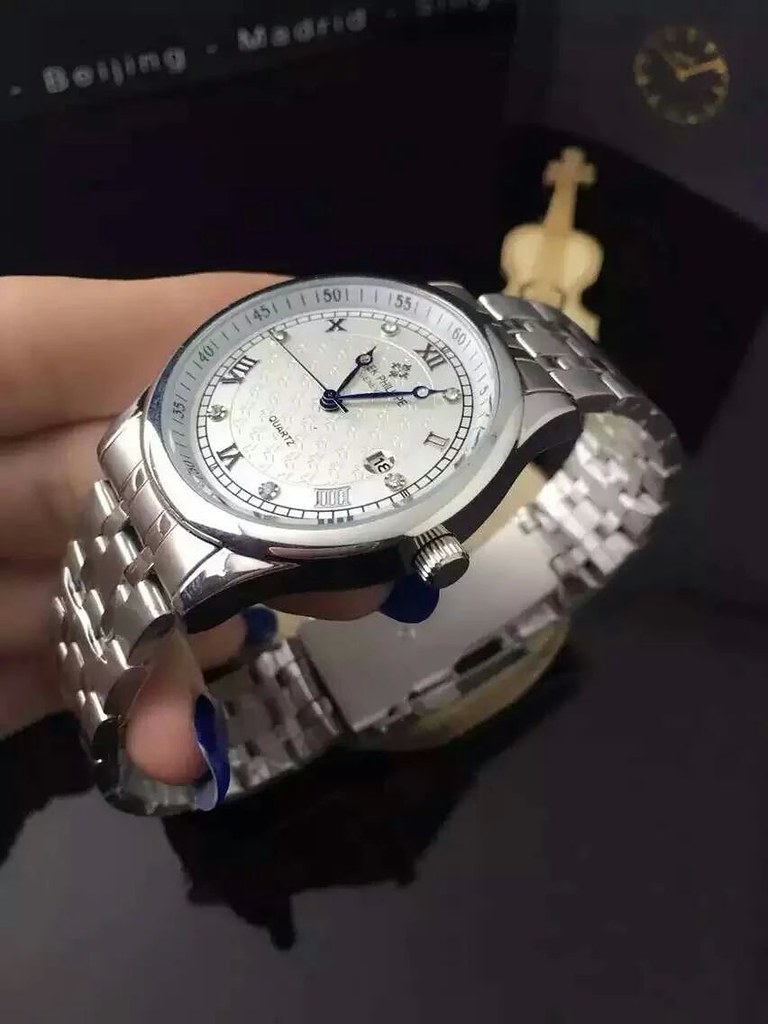A person holds a stainless steel watch in their left hand, prominently displaying the intricate details of the timepiece. The watch face features classic Roman numerals at the 12, 2, 4, 6, 8, and 10 o'clock positions, each slightly raised for a distinguished look. The dial showcases the name "EK Philippe," suggesting a possible Patek Philippe, a renowned luxury watch brand, although the full brand name is partially obscured. Just above the branding, a delicate insignia resembling a cross with leaf-like extensions adds an elegant touch, though its exact design is difficult to discern.

The watch indicates the time as 11:05, with the second hand precisely pointing at the 45-second mark. It is a quartz watch, featuring a date display showing the 18th of the month. A winder is also visible, and the seconds are marked from 5 to 60 in five-second increments around the edge of the dial.

This sophisticated timepiece is held over a gleaming black surface, possibly a lacquered table, reflecting the watch and the holder's hand. Additionally, a faint outline of a gold violin can be spotted in the background, adding an artistic and luxurious context to the scene.